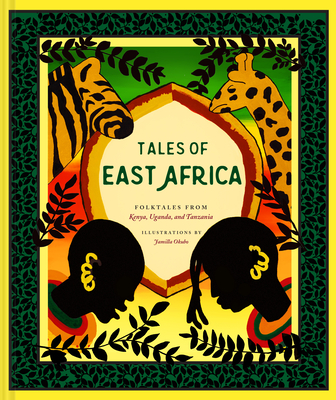The image is a vertical rectangle resembling the cover of a book titled "Tales of East Africa." The book is surrounded by a thin yellow border, followed by a thicker green border decorated with black leaves. Within this, there's a light yellow border framing the actual cover design. The cover is divided into two main sections: the upper fourth is green, while the lower three-fourths is yellow. At the top left corner, there's a zebra with black stripes on a yellow body, and at the top right corner, a similarly colored giraffe with black spots. 

In the center, there is a shield-shaped icon bordered in yellow and red, containing white space with the title "Tales of East Africa" in green text. Below the title, it reads "Folktales from Kenya, Uganda, and Tanzania," though this text is somewhat blurry. Further below, it mentions an illustrator’s name in red text. In the bottom section of the cover, two black silhouetted heads face downward towards the center; each figure has yellow earrings and is adorned with multi-layered necklaces featuring orange, green, and red hues. Silhouetted vines and leaves fill the remaining space on the bottom, with additional leafy branches appearing on both sides.